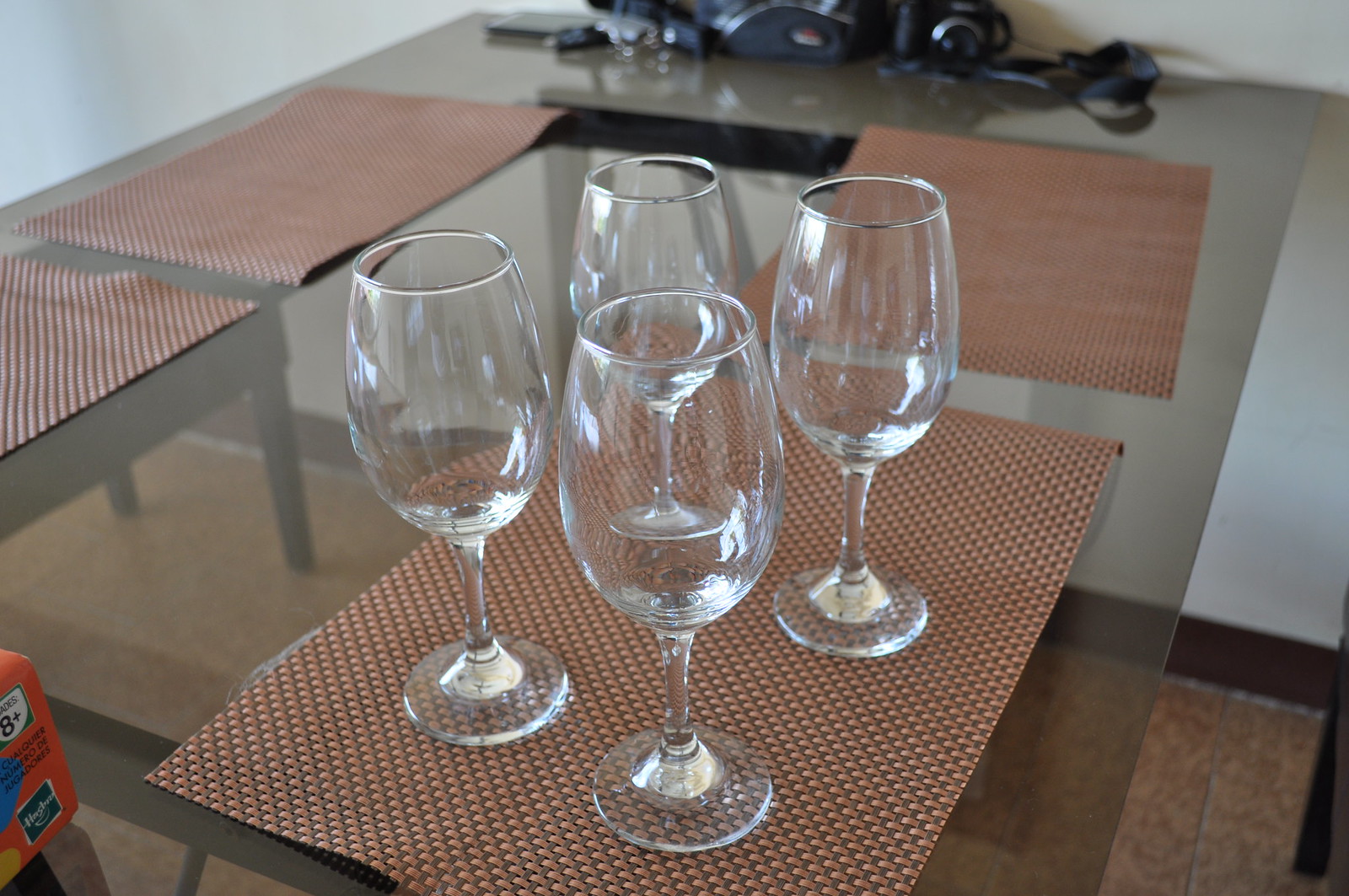The image depicts an indoor scene featuring a glass table situated on a light reddish tiled floor. The table has a transparent surface and is accompanied by a brown border towards the back. On the table, there are four burgundy-colored placemats, one of which, positioned at the front right, holds four empty wine glasses arranged neatly in a two-by-two square. Additionally, there's an orange container with the number 8 and a green label, located at the bottom left corner of the table. In the background, several out-of-focus objects, possibly camera equipment or metallic items like keys or bottle openers, are seen on the back end of the table. The backdrop includes a white wall with a brown baseboard at the bottom.